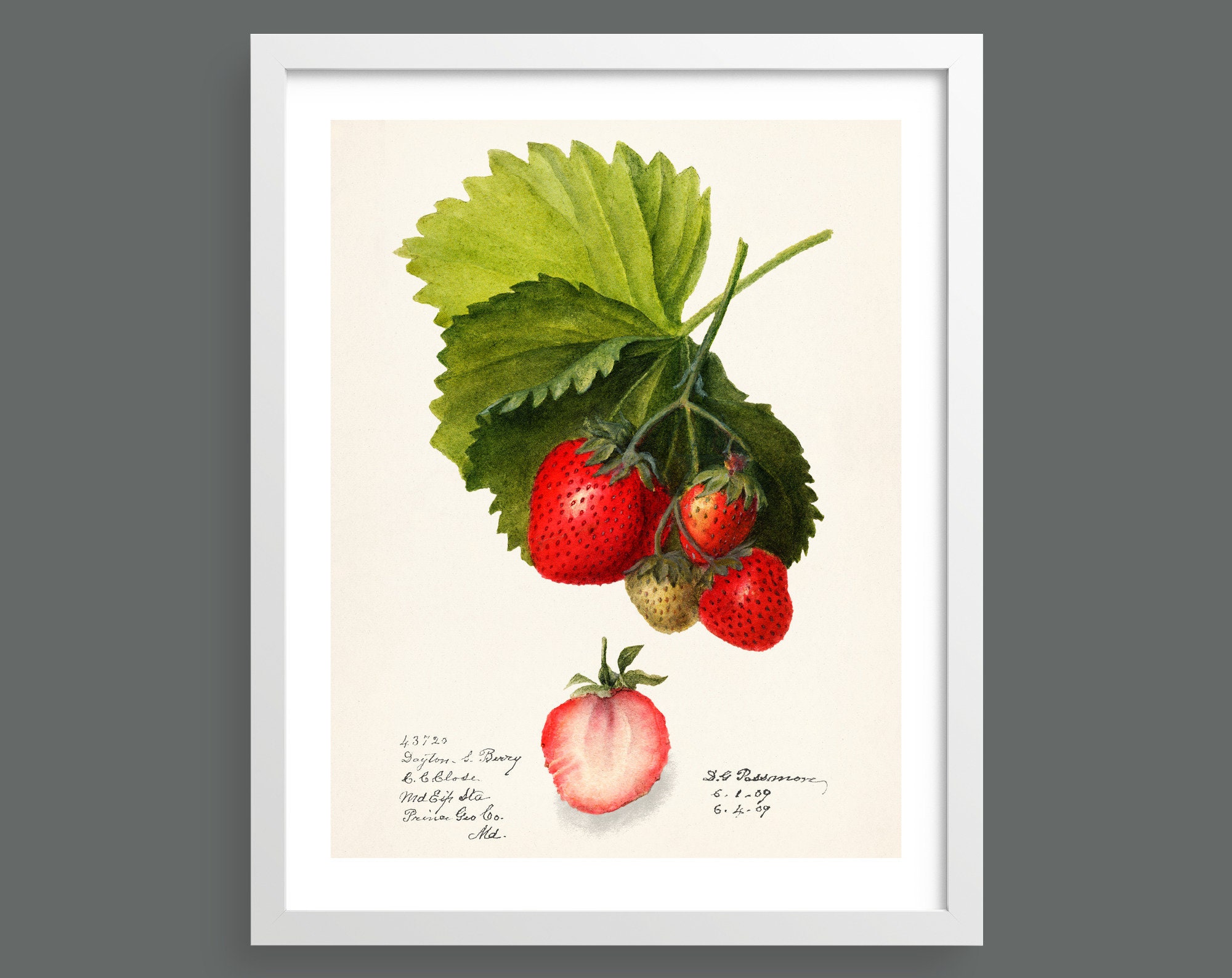The framed painting hanging on a dark gray wall features a detailed color illustration of a cluster of strawberries rendered in what appears to be colored pencil. The artwork is set inside a light gray frame with a light tan background. At the center of the painting, a bunch of strawberries hangs from their stem, surrounded by broad, ridged green leaves that fan out behind them. Among the vibrant red strawberries, one still remains light green, indicating it is not yet ripe. Additionally, there is a cross-section of a strawberry, sliced in half to reveal its interior, positioned near the bottom of the illustration. The image includes small, unreadable cursive writing and signatures on the left and right, possibly including dates. The attention to detail in the textured seeds and the naturalistic depiction of the strawberries makes this painting both realistic and aesthetically pleasing.